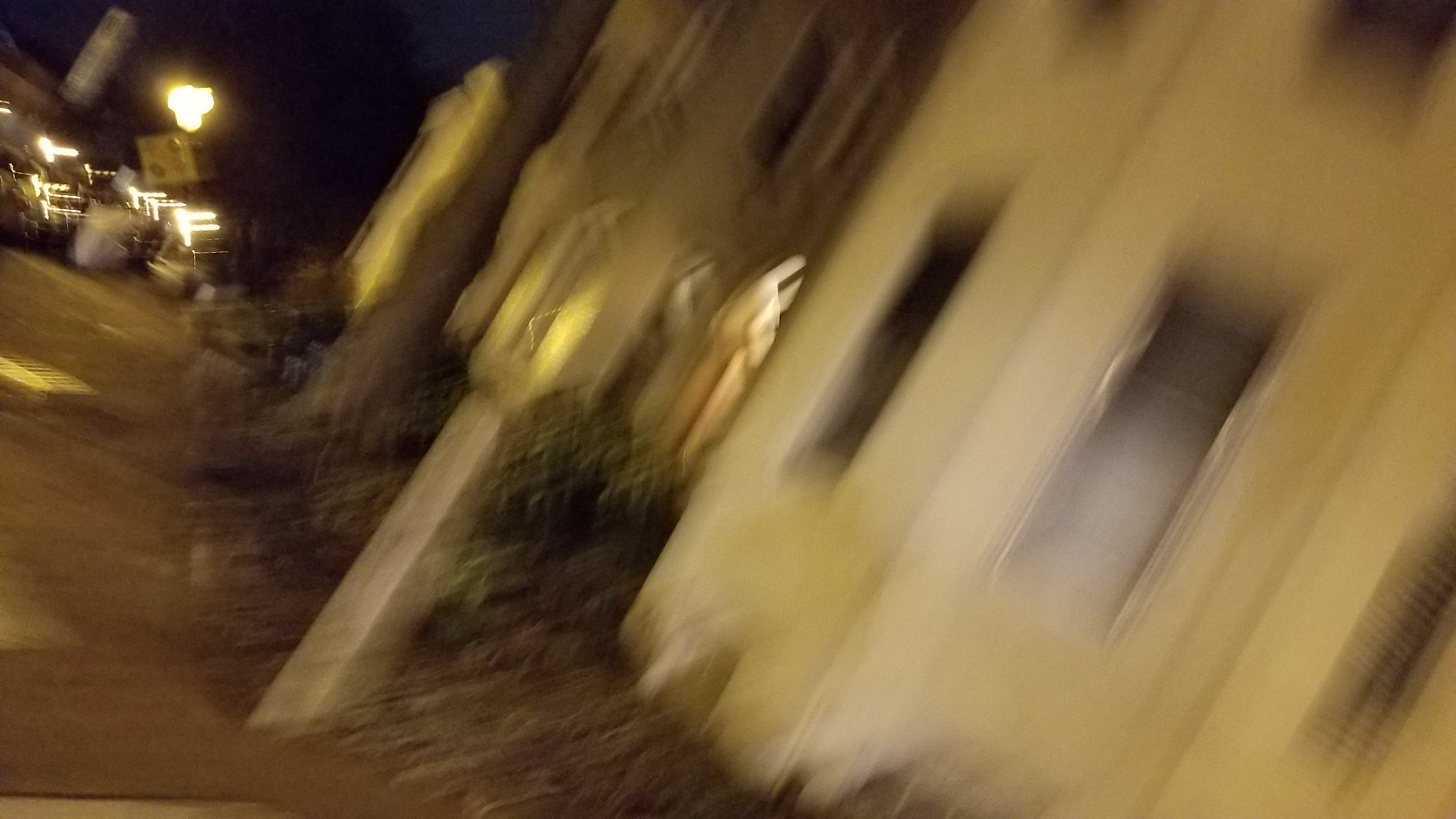This photograph is an extremely blurry outdoor shot taken at an angle, making the scene appear tilted, as if the buildings within it are leaning sideways or falling backward. The central focus seems to be a cream-colored or white building, possibly a house or an apartment, characterized by elongated or narrow windows. There are about three windows visible on this structure. To the right, there's another building with windows and some greenery, possibly shrubs or bushes in front. A distinguishable feature of the main building is the presence of round columns at its front, along with another column on the side.

The foreground seems to feature what could be a yard or driveway that appears distorted due to the camera angle. Additionally, towards the left and the top of the photograph, several lights are visible, although their sources are indiscernible. There's also a noticeable yellow diamond-shaped sign with reflectors on it, which could be a street or construction sign, though its text is illegible. The overall image is very jagged and out of focus, complicating the clarity of the scene.